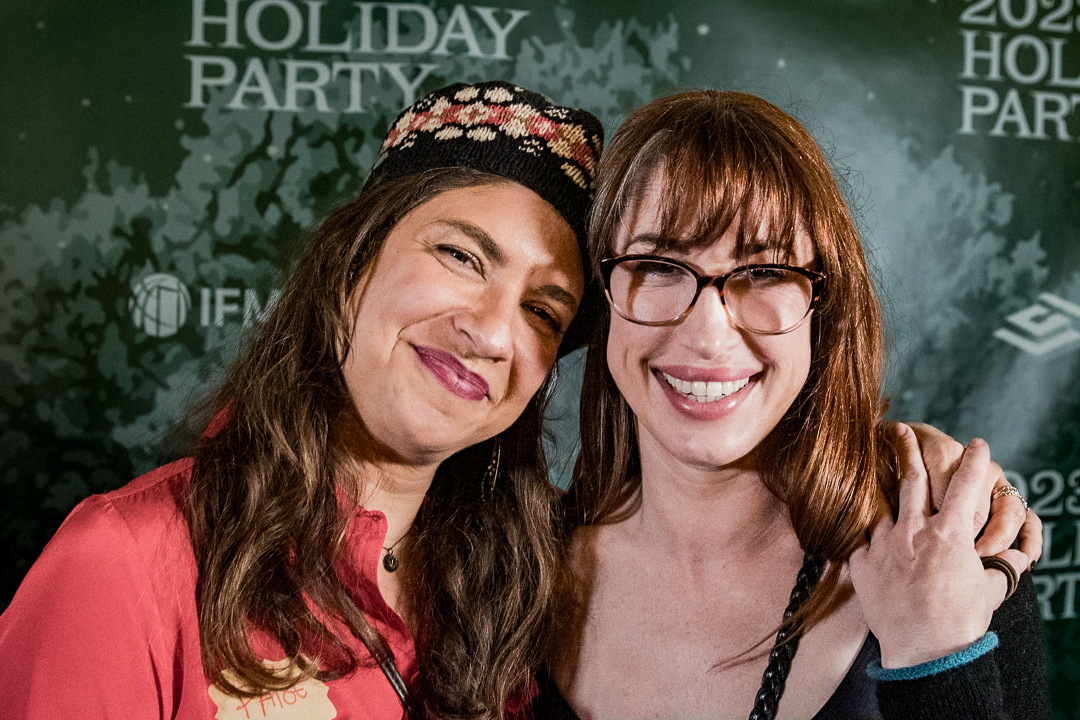This vibrant and cheerful photograph, taken at a 2023 Holiday Party, features two women in their early 40s standing in front of a green backdrop adorned with the IFM logo, which features a spherical earth design. The backdrop also prominently displays "Holiday Party" in white lettering. The woman on the left is characterized by her wavy dark brown hair cascading past her shoulders and her colorful ensemble, which includes a bright pink jacket and a knitted hat with red, black, and white polka dots. She'd likely be seen smiling softly with her eyes slightly closed and adorned with pink lipstick, a yellow name tag with "Payote" in red, a black necklace, and a brown strap across her chest. The woman on the right is dressed in a black sweater with a blue bottom rim around her wrist and wears black-framed glasses that have brown accents. Her striking burnt auburn hair and beaming, toothy smile add to her welcoming appearance. Both women are engaged in a warm, friendly pose, with the woman on the right placing her hand around her companion's shoulder, signifying a strong camaraderie and festive spirit.